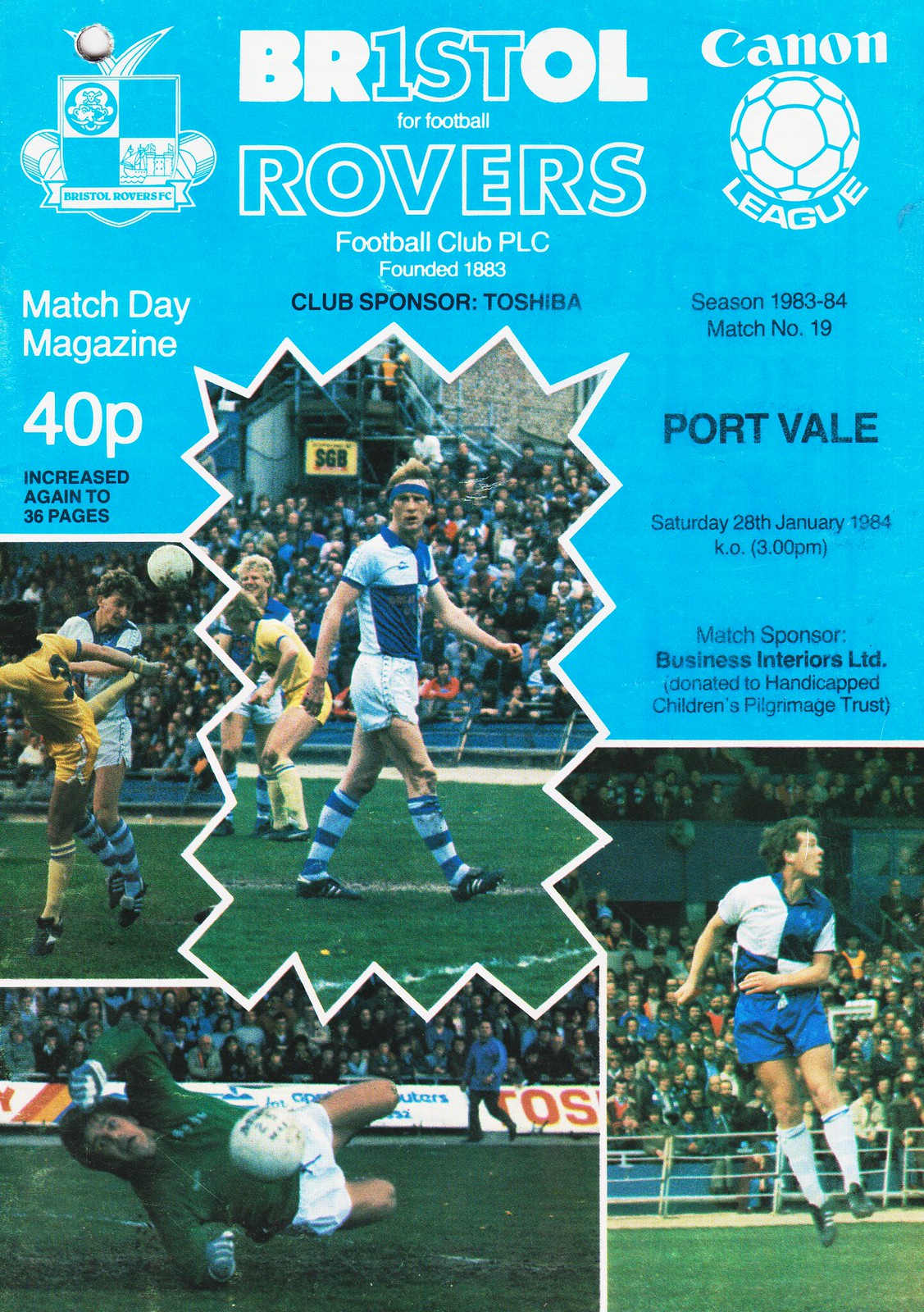This is a detailed advertisement or poster for a soccer event featuring the Bristol Rovers FC. In the upper right-hand corner, there is a "Canon League" title with a white soccer ball situated between the words. In the upper left-hand corner, a square logo of the Bristol Rovers FC is displayed, designed as an upside-down shield which includes two blue squares and two white squares with images inside. Across the top of the flyer, it prominently states, "Bristol for football Rovers Football Club PLC, Founded 1883. Club Sponsor Toshiba." The "Bristol for" part interestingly replaces the 'I' in Bristol with a '1', emphasizing "Bristol 1st."

To the left side of the poster, it mentions, "Match Day Magazine 40p, Increased Again to 36 Pages." Central to the design are four photographs showcasing soccer players actively engaged in the game. To the right of these images, it indicates, "Season 1983-84, Match Number 19." Below this, it specifies the match details, "Port Vale, Saturday 28th January 1984. KO 3 p.m." Additionally, it notes the match sponsor, "Business Interiors Limited," with a special mention that it is, "Donated to Handicapped Children's Pilgrimage Trust." The backdrop of the entire poster is in a light blue color, enhancing the visibility of the detailed information and varied visual content presented.